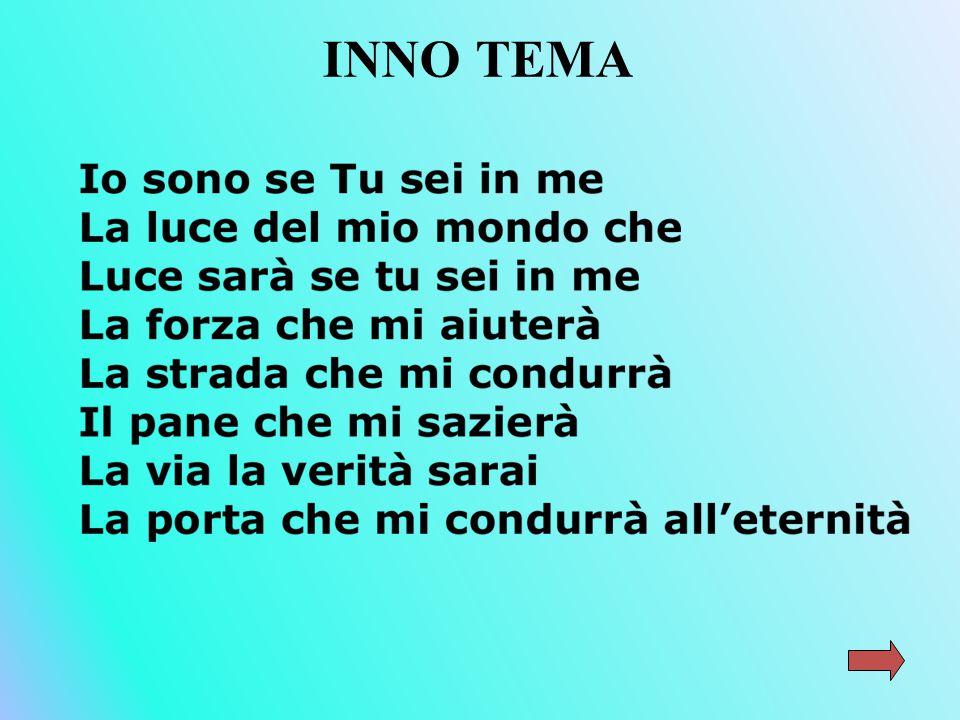The image features a square with a light teal background that gradually shifts to light blue from the bottom left to the upper right. Prominently displayed in black text at the top center are the words "Ino Tima." Beneath this heading, there are several lines of text in a foreign language, starting with "Io sono se tu sei in me," followed by "La luce del mio mondo e che," "Luce sara se tu e si in me," "La forza che mi atoria," "La strada che mi candura," "Il pen che mi sazeria," "La via la vertia sarai," and finally, "La porta che mi candura al eternitira." At the bottom right corner, there is a noticeable red arrow pointing to the right. This cropped snapshot likely originates from a website, displaying only the text on a powder green and blue gradient background without any additional web interface elements, date, or time.